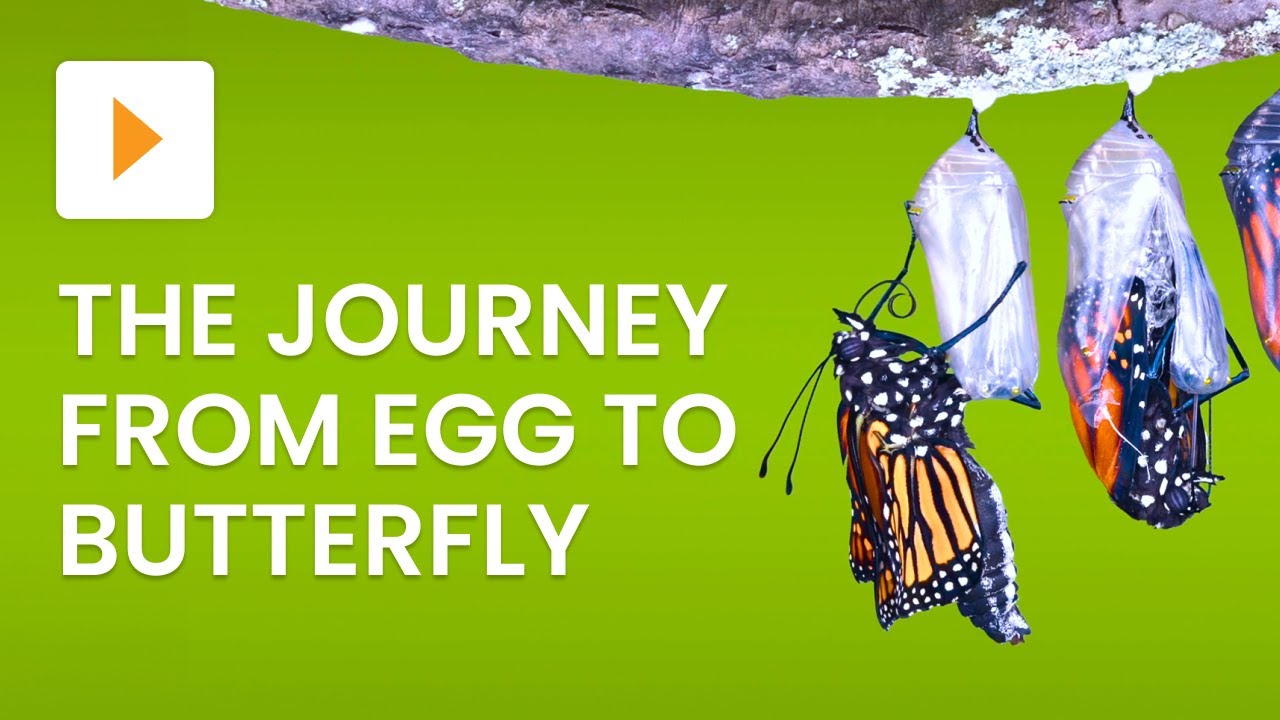The digital poster features a striking image of a butterfly hanging from its empty cocoon, which is cream-colored and prominently positioned on the right side. The butterfly, recently emerged, showcases its stunning black body adorned with white spots and vibrant orange and black wings, offering a sharp contrast against the blurred green background that hints at an outdoor setting. On the left side of the poster, bold white capital letters read "LIFE CYCLE OF A BUTTERFLY," centrally placed from top to bottom. Above this text on the left, there's an icon featuring an orange triangle, resembling a play button, set within a white square. The blend of natural elements and textual information vividly illustrates the metamorphosis of the butterfly, capturing both the beauty and the transformative process of its life cycle.